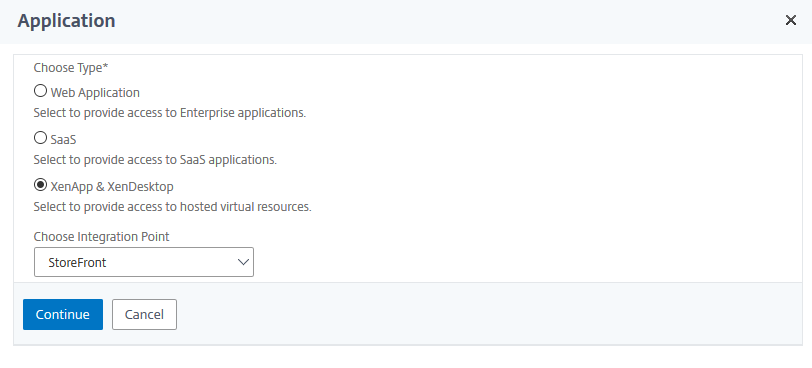This image is a simple user interface screenshot featuring a predominantly white background with minimalistic design elements. The screen is primarily composed of text boxes, standard buttons, and radio buttons, all of which are left-aligned, contributing to a clean and uncluttered look with ample white space. 

At the very top of the screen, there is a gray banner displaying the title of the application. On the far right of this banner, there is an "X" button used to close or exit the screen. Below the banner, the user is prompted to "choose type," offering three distinct radio button options:

1. **Web Application**: Select to provide access to enterprise applications. 
2. **SAAS (or SaaS)**: Select to provide access to Software as a Service applications.
3. **ZenApp and ZenDesktop**: This option, which is already selected, allows the user to provide access to hosted virtual resources.

Underneath these options, there is an additional choice to "choose the integration point," with the selectable option being "storefront."

Notably, the font is black, contrasting sharply against the white background, enhancing readability. There are a few gray banners and a prominent blue button that stands out on the otherwise plain interface.